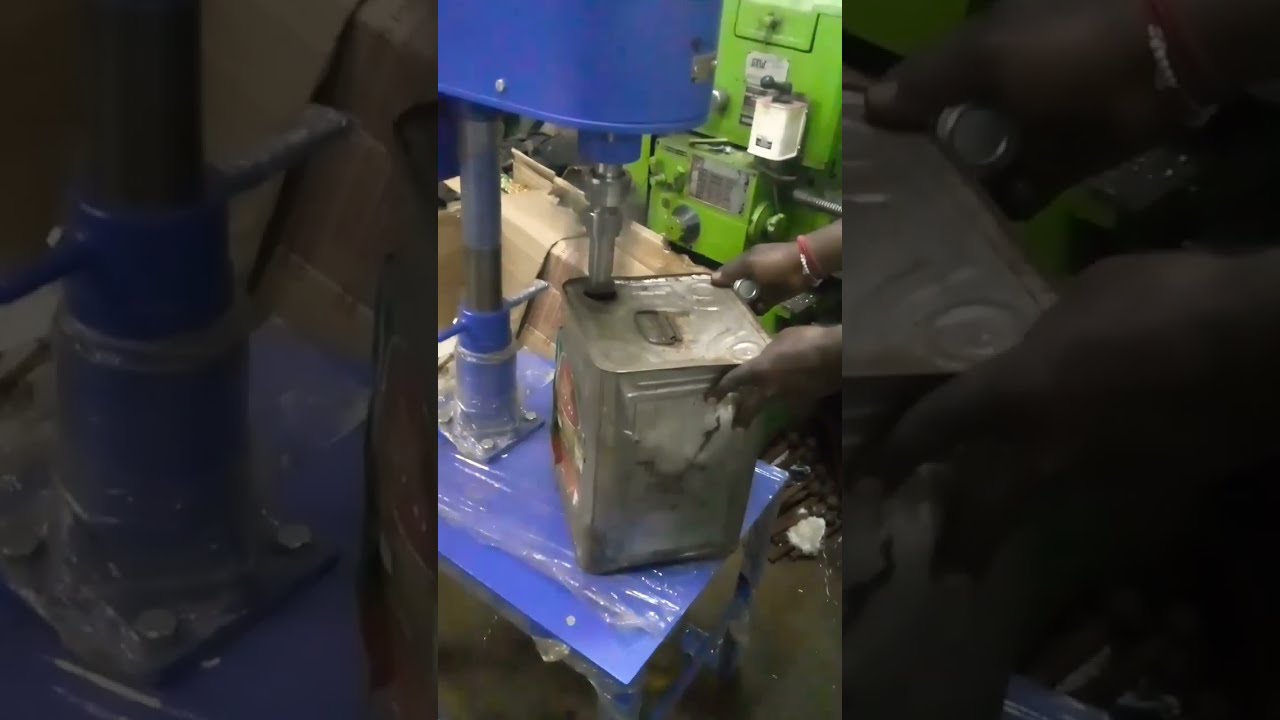The image depicts a scene from an indoor mechanic or machine shop, emphasizing a vertically aligned photograph reoriented into a horizontal format, resulting in two added black panels on the sides. 

In the left segment, a dark blue-colored conical device, connected perpendicularly by a circular metal rod and possibly secured by a vice, is prominently shown. This blue cylinder connects to a metal plate at the bottom with several thick screws, suggesting a sturdy setup. Behind this apparatus, there are brown wooden walls on the upper left and upper right.

The central part of the image provides an expanded view; the blue cylinder device is visible at the edge, and a large rectangular metal tin can is being held upright by two hands on a light blue table. A thick metal drill appears to be piercing or interacting with the tin can from above, illustrating some form of metalworking or drilling process. The background here reveals a light green wall, another piece of industrial equipment, and several cardboard boxes.

The right segment of the image captures a close-up of the two hands, now holding what seems to be the cap of the metal tin can, further implying that the machine might have been used to remove the top of the tin can. The background in this section features dark brown and green hues with various unidentifiable supplies.

Overall, the photograph showcases detailed machine shop activity, involving a blue stationary drill or clamp device interacting with a metal container, with additional machinery and equipment in the surroundings.